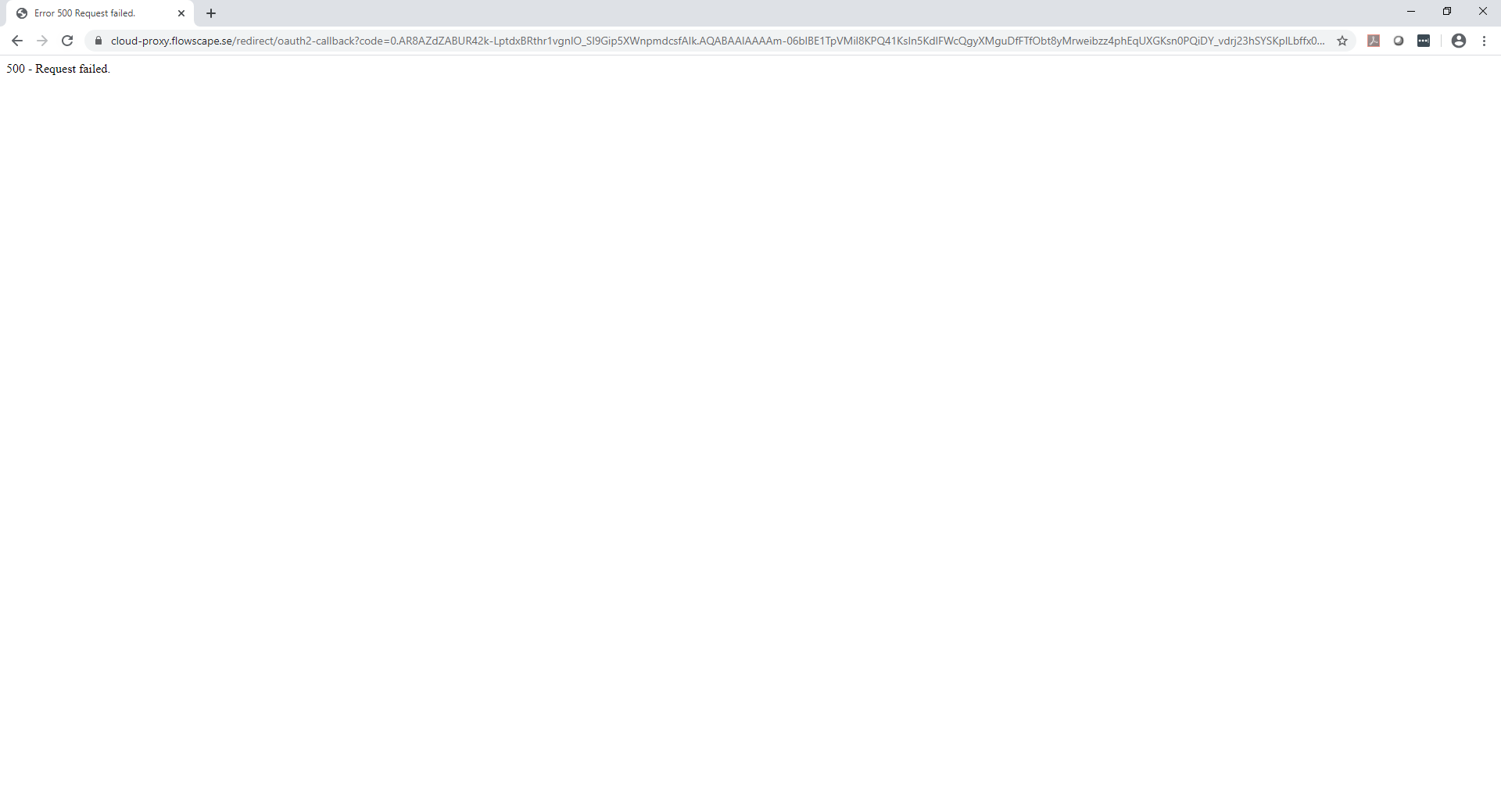This is a detailed image description for a screenshot that contains minimal but critical information:

The screenshot captures an error message in a web browser window. The top of the browser window shows a white tab containing a globe icon, followed by the text "error 500 requests failed" in black font and a black X on the far right. The browser’s address bar is split into two main sections: the left portion features a thin gray bar with a black plus arrow on the far left, and a black square with a black X on the far right. 

Below this section, against a white background, there are navigation buttons: a black back arrow, a gray forward arrow, and a black reload button. The URL bar stretches across the screenshot, displaying a very light gray background with a dark gray padlock icon on the left. The URL starts with "cloud-proxy.flowscape.se" in black text and spans the entire width of the image. At the right end of the URL bar, there is a star icon for bookmarking, followed by a small square, a circle, a black square with three white horizontal dots, a user icon in gray depicting a human shape, and finally, three vertical dots.

At the bottom of the white background, the text "500-request-failed" is displayed, indicating the error message. The overall image is sparse and challenging to read, with very small print that remains unclear even when enlarged.